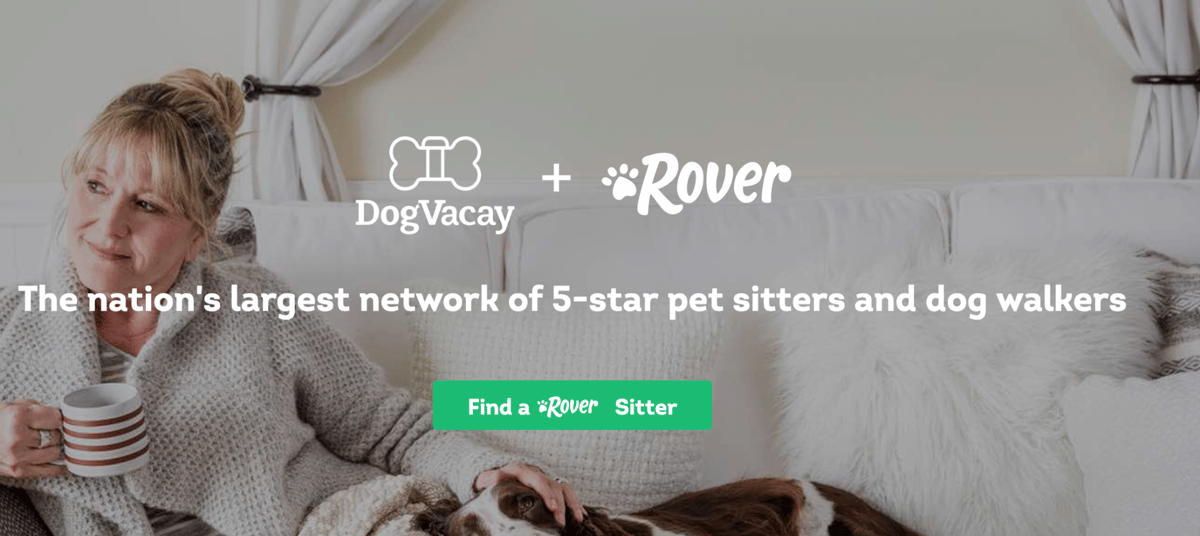Sure, here's a cleaned-up and detailed caption for the image:

---

The promotional image highlights a partnership between DogVacay and Rover, two prominent pet care services. A woman, comfortably seated on a light-colored sofa, is dressed in a cozy gray sweater and holds a white mug adorned with red and brown stripes. Adjacent to her on the sofa is a relaxed brown and white dog, exuding comfort and calm. 

At the top center of the image, the DogVacay logo, featuring a bone icon, and the Rover logo, showcasing a paw print, are displayed side by side with a plus sign in between, symbolizing their collaboration. Beneath the logos, bold white text proclaims, "The nation’s largest network of five-star pet sitters and dog walkers." 

A prominent green button at the bottom of the image, with the text "Find a Rover Sitter" in white, invites action. The overall warm and homey aesthetic of the image effectively conveys the sense of comfort and care that both DogVacay and Rover seek to provide through their services.